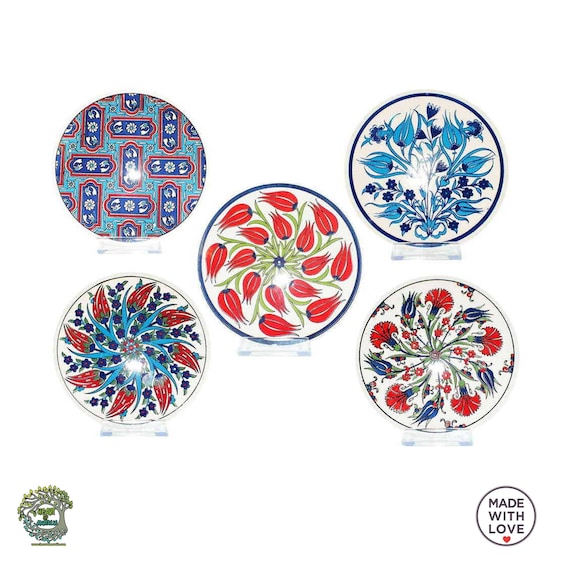The image is a color illustration of five vertically held ceramic plates, each set in glass or plastic holders against a white background. The plates feature various floral and plant-themed patterns in prominent colors of red, blue, and occasionally green. The patterns include intricate designs with flowers, leaves, and plant-like motifs. One plate stands at the center displaying a green plant with red bulbs, while another in the lower left showcases blue leaves and red flower buds in a circular arrangement. There is also a plate in the upper left corner with a repetitive rectangular pattern, different from the others in its abstract design. In the bottom right corner, a circular logo reads "MADE WITH LOVE" in black capital letters, accompanied by a small red heart. Another logo in the bottom left corner depicts a tree, although the accompanying text is unclear. The arrangement is two plates on top, two on the bottom, and one in the center, all reflecting light, indicating their ceramic nature.